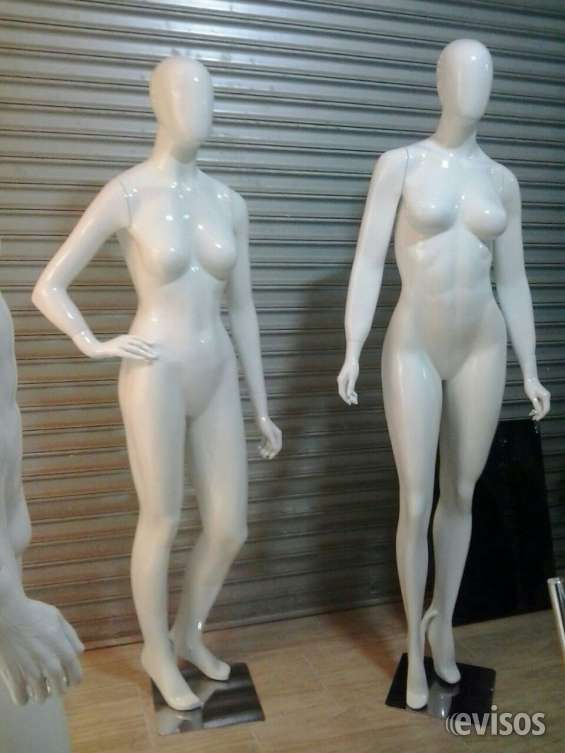The photograph depicts a storefront with a closed, metallic gate resembling a garage door, featuring three glass-like mannequins. Dominating the image are two unclothed female mannequins standing on square, mirrored bases against a backdrop of wooden panel flooring. Both figures stand on their tiptoes, seemingly imitating the posture of wearing high heels. Positioned on the left, one mannequin strikes a pose with her left hand on her hip while the right arm hangs down. The mannequin on the right, whose head is slightly cut off from the frame, stands with both arms straight at her sides and one foot in front of the other. A third mannequin, partially visible on the far left side of the image, appears to have a muscular male torso, with its right hand in view. The only text present in the image is the word "EVISOS," situated in the bottom right corner.